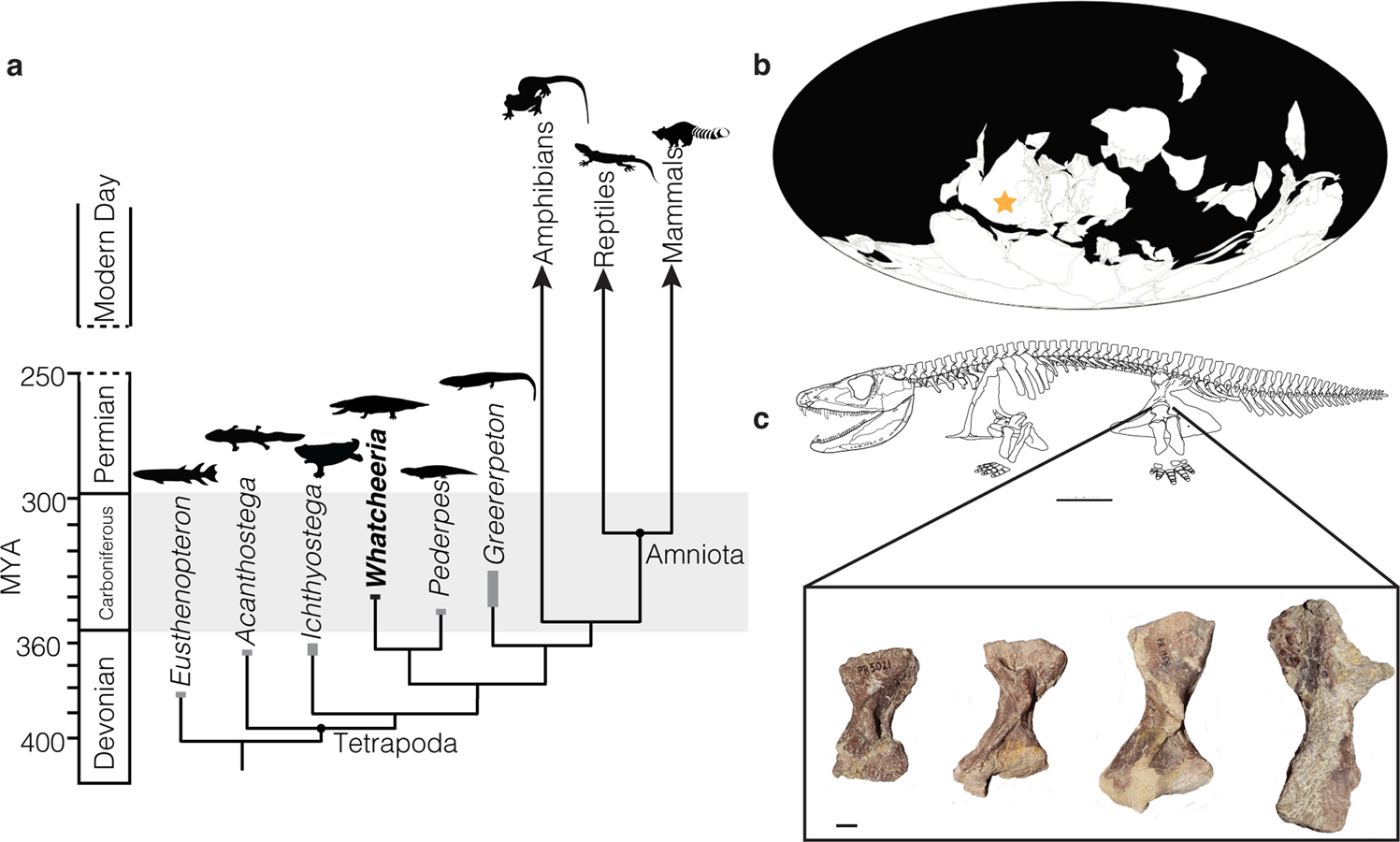The image is an informative chart detailing the evolution of reptiles through various geological eras. On the left-hand side, labeled as section A, there's a chronological graph depicting time from the Devonian period (around 400 million years ago) through the Carboniferous (circa 360 million years ago) and the Permian (up to 250 million years ago), ending at Modern Day. The chart categorizes various species with their scientific names, positioned according to their respective eras. Among these, illustrations of fish, amphibians, reptiles, and mammals are placed at different elevations on the chart.

In the upper right-hand corner of the image, labeled as section B, is a black-and-white, oval-shaped map of the Earth with a yellow star indicating the location, possibly Australia, where the fossils were discovered.

Section C, on the lower right side, features the profile view of a prehistoric reptile's skeleton. Highlighted within this skeleton are specific areas linked to actual photographs of four fossilized bones. These bones vary in size, lying from smallest to largest, and are displayed in a sequential manner beneath the skeletal drawing. The comprehensive layout illustrates both the evolutionary timeline and the physical evidence supporting the study.